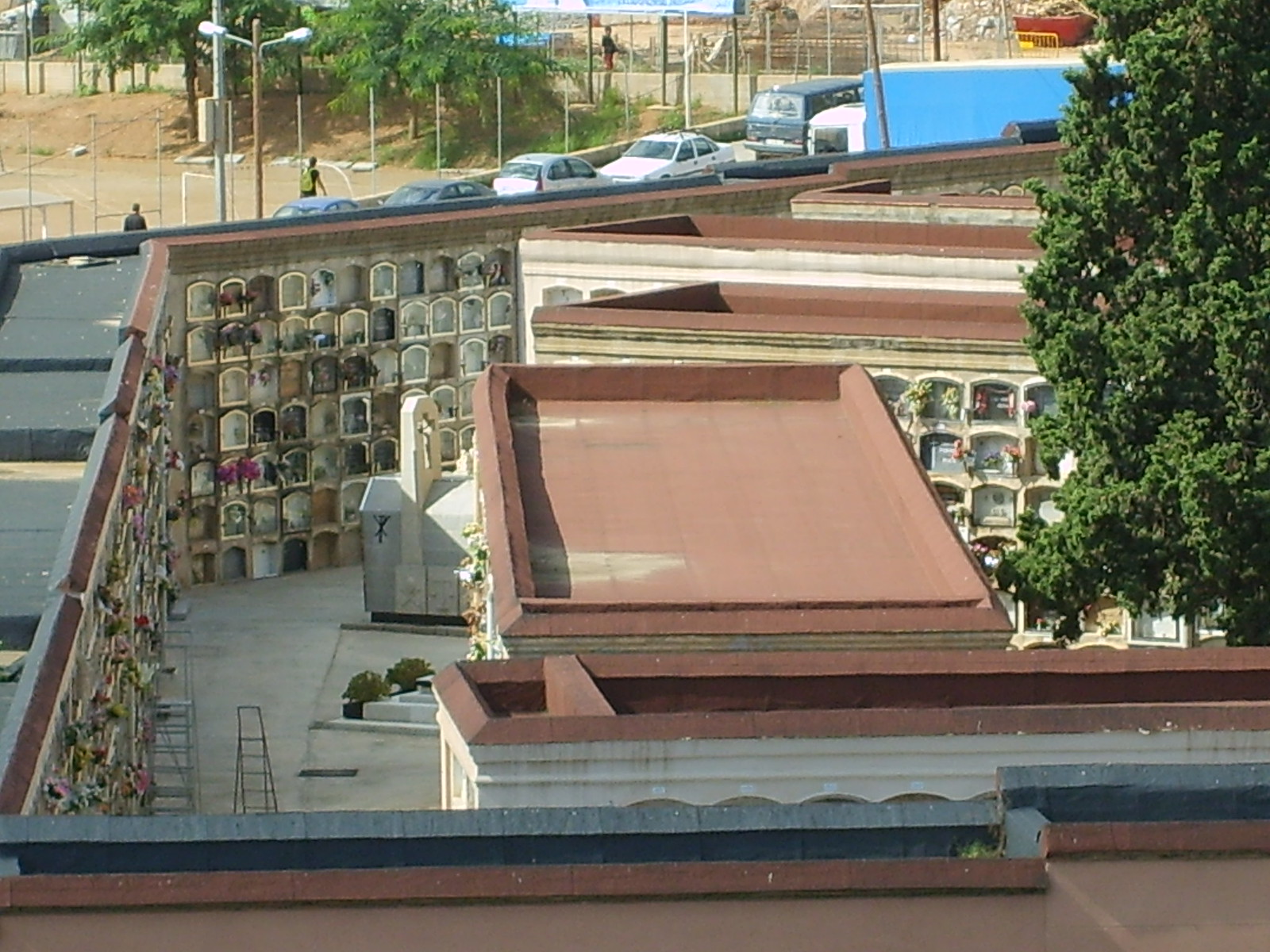The photograph is taken from an elevated position, perhaps the roof of a building, capturing a view of an unusual grave site that resembles an open-air courtyard. The prominent colors in the image are green from the few trees and brown-red from the roof tiles. The courtyard is surrounded by high walls and contains multiple tombstones, suggesting it's part of a mortuary. Inside the fenced area are various containers, their contents indistinct, contributing to the industrial urban feel of the environment. The image appears to be from an older era, around the mid-1970s, indicated by the style of the cars parked along a road and visible trucks. There are a couple of people in the scene, one of whom is carrying a backpack. Streetlights and a sparse scattering of greenery further characterize the setting.